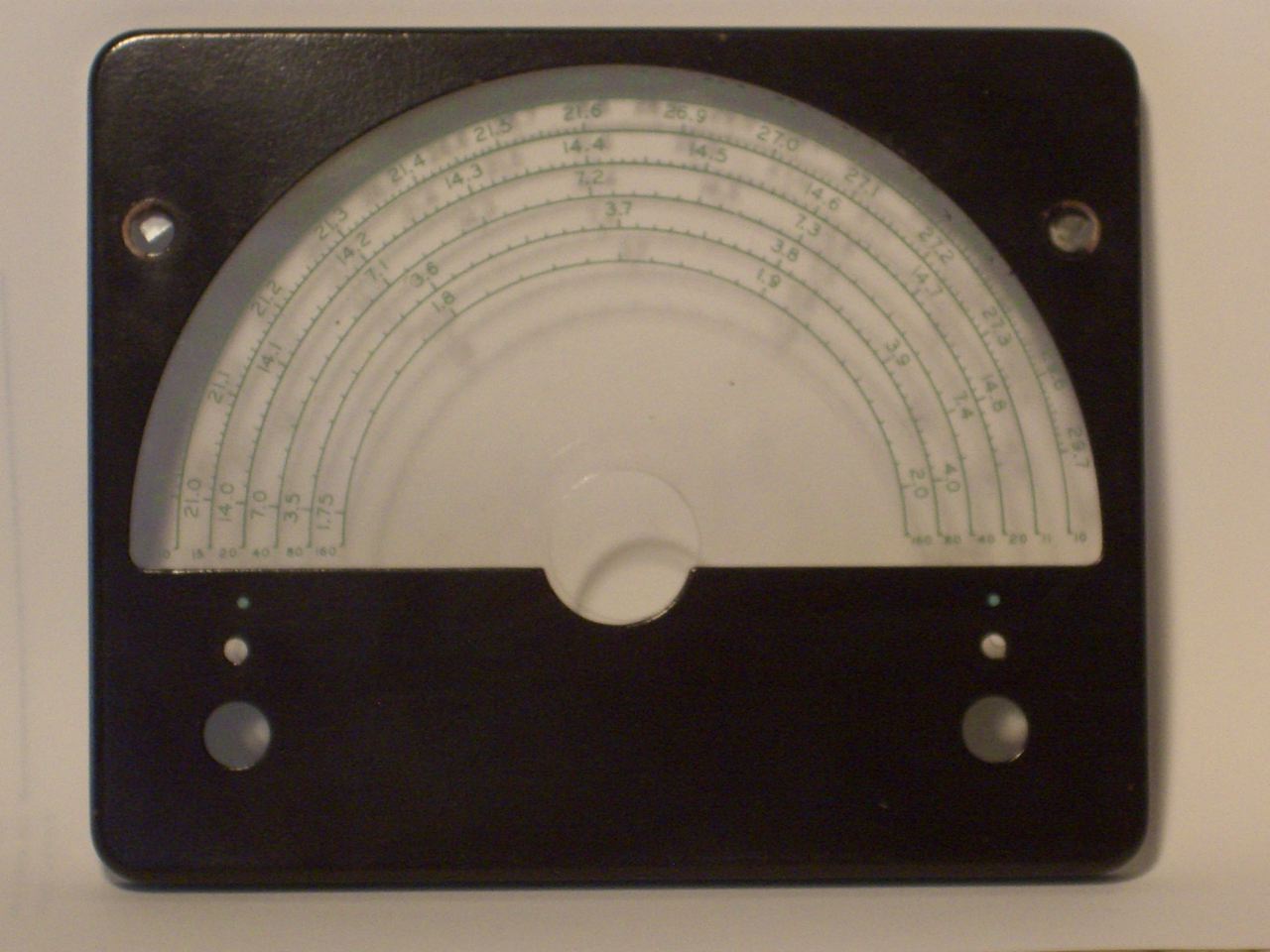This image showcases a semi-circular protractor commonly used in mathematical and geometric work. The protractor resembles the arc of a rainbow, characterized by five thin, green, concentric lines that form its shape. From the left corner, there are numerical labels: 21.0, 14.0, 7.0, 3.5, and 1.75, sequentially decreasing vertically. These numbers mark the measurements which are further extended along the green lines that radiate outward.

Additionally, there are small vertical lines placed at intervals along these concentric lines, accompanied by further numerical annotations. At the center of the protractor, the value 21.6 is clearly indicated, which progresses to 27 on the right side. 

Surrounding this protractor, there are four black circular tabs, each about half an inch in diameter, positioned on a flat black piece. Below the protractor, there is a white turning knob shaped like a semi-circle, presumably to adjust or rotate a part of the protractor.